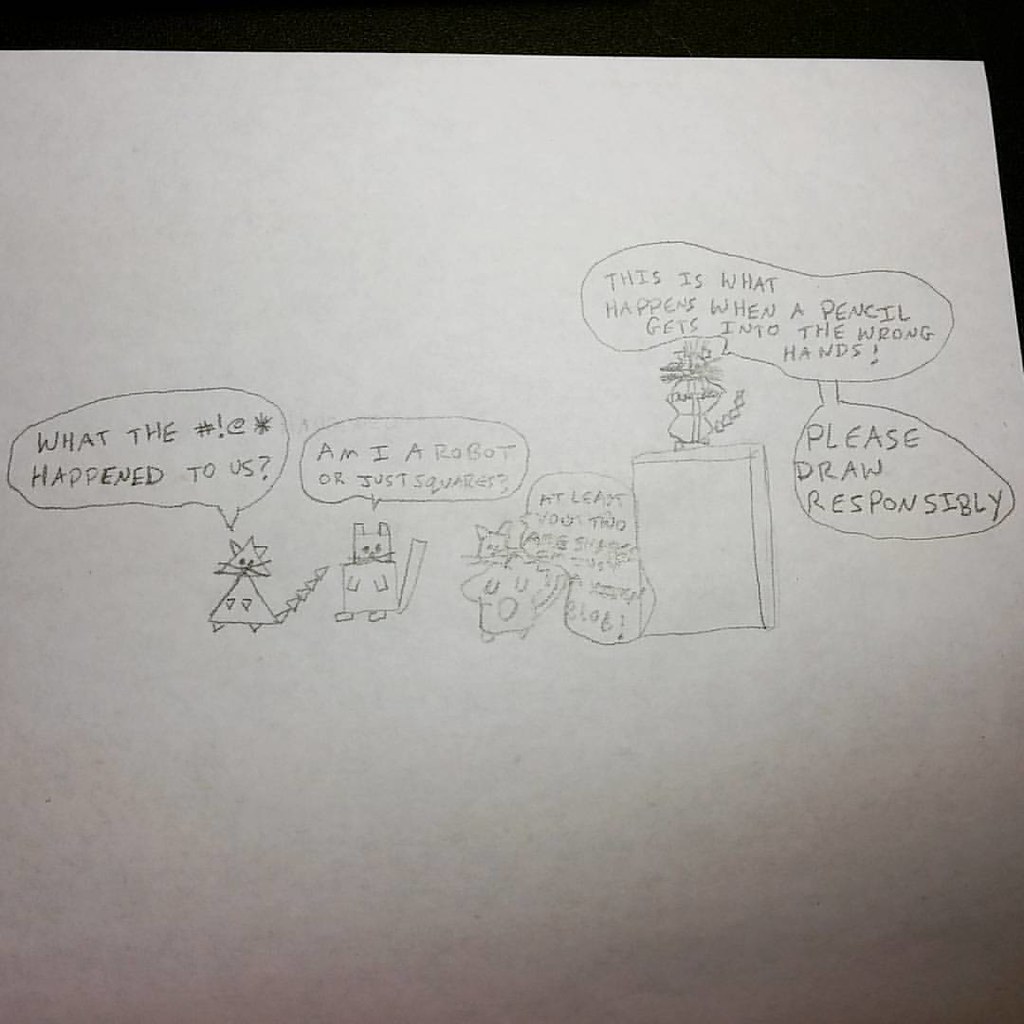The image depicts a detailed cartoon drawing on a white piece of paper with a black background. Central to the image are characters styled as cats, each drawn with different shapes and each appearing in a row. On the left is a triangular cat with a thought bubble reading, "What the #@*! happened to us?" Next to it, a rectangular cat's thought bubble says, "Am I a robot or just squares?" Following that, a squiggly, blob-like cat expresses in its thought bubble, "At least you two are shapes, I'm a blob." On the far right, a cube with another cat perched on top has a thought bubble stating, "This is what happens when a pencil gets into the wrong hands. Please draw responsibly." All the text and figures are rendered in black or gray, presumably in pencil, against the stark white background of the paper.